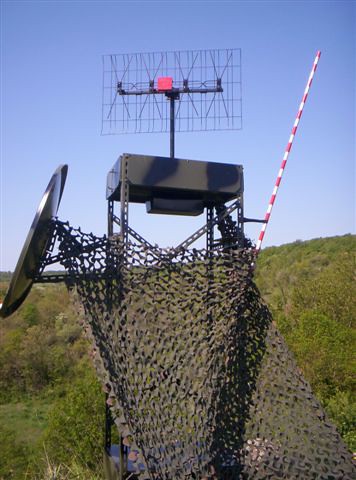In this detailed outdoor photograph, we're looking at a metal antenna tower situated against a backdrop of lush green forest and a vibrant clear blue sky. The tower, blackish-gray in color, rises prominently above the surrounding shrubs and greenery. Attached to the left of the tower is a large, brushed silver satellite dish pointing left. On the right side of the tower, there's a distinct red and white striped pole angling upwards. The antenna array at the top of the tower features a square gray metal frame with crossed wires and houses a small red box. The structure descends to the ground, supported by green square poles. Notably, there is an extensive green mesh that stretches over part of the tower, contributing to its somewhat camouflaged appearance. This mesh extends from the satellite dish and attaches to various points on the tower, creating an intricate and visually striking scene against the natural and serene background.